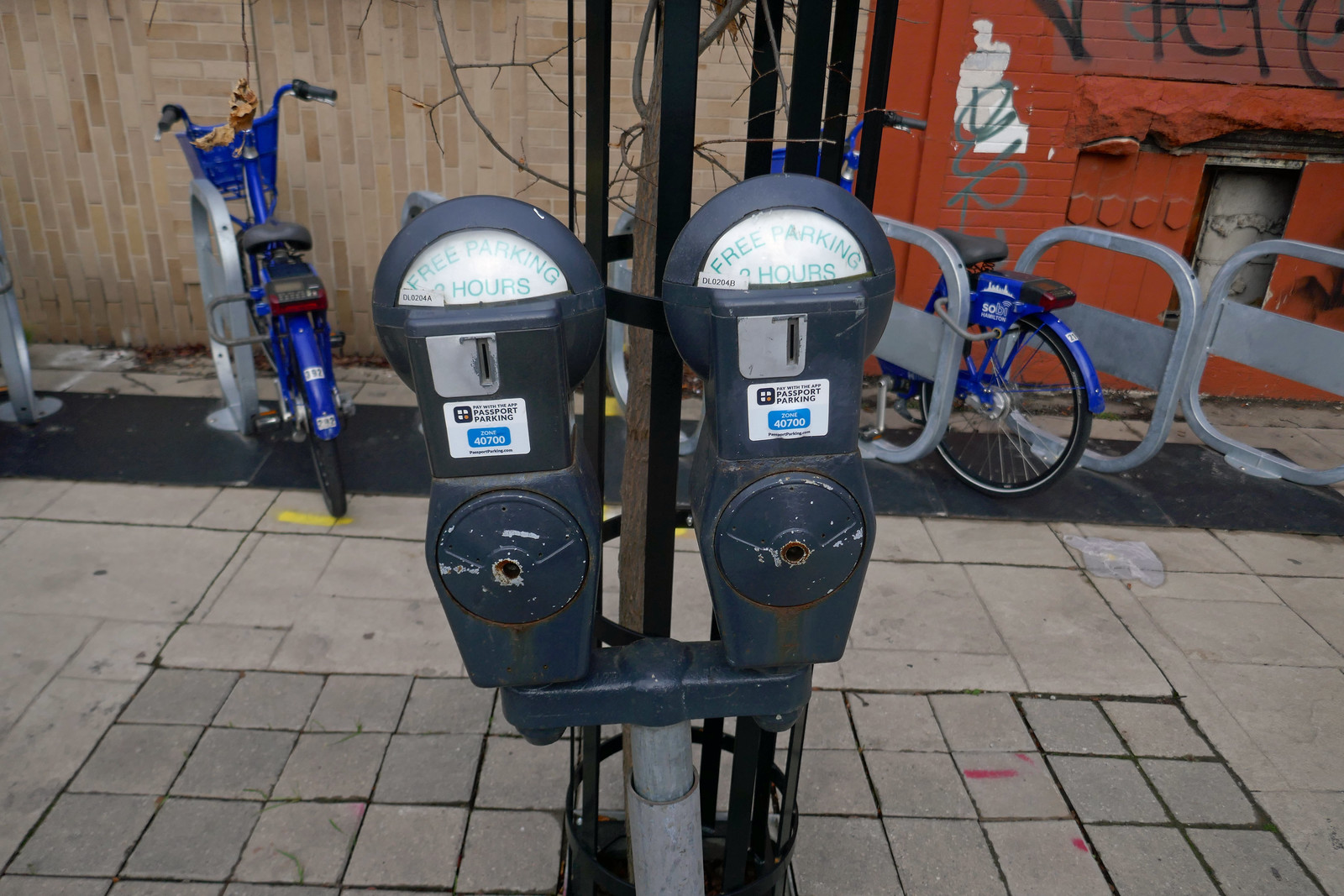In this highly detailed image, we observe two parking meters prominently positioned at the forefront. These meters are painted a dark bluish-gray color and are mounted on gray poles. Each meter features a coin slot in silver and bears multiple labels. Up top, the text "Free Parking Hours" is clearly visible, written in a light bluish font against a white background. Another sticker on the meters reads "Passport Parking Pay with the App," including the zone number 4700 and additional digits such as 407090 and L020431.

In the background, a variety of elements add depth to the scene. A silver metal bike rack holds identical blue bicycles, locked securely with gray locks. The backdrop includes two buildings: the left one is a mix of vertically and horizontally arranged bricks in browns, grays, and whites, while the right building is shaded in orange-brown hues and is covered in graffiti. Additionally, there is a silver metal fence that adds to the urban setting. The ground is constructed of concrete with sporadic red and yellow markings. The entire scene is captured in daylight, amplifying the vivid colors and intricate details of this urban milieu.